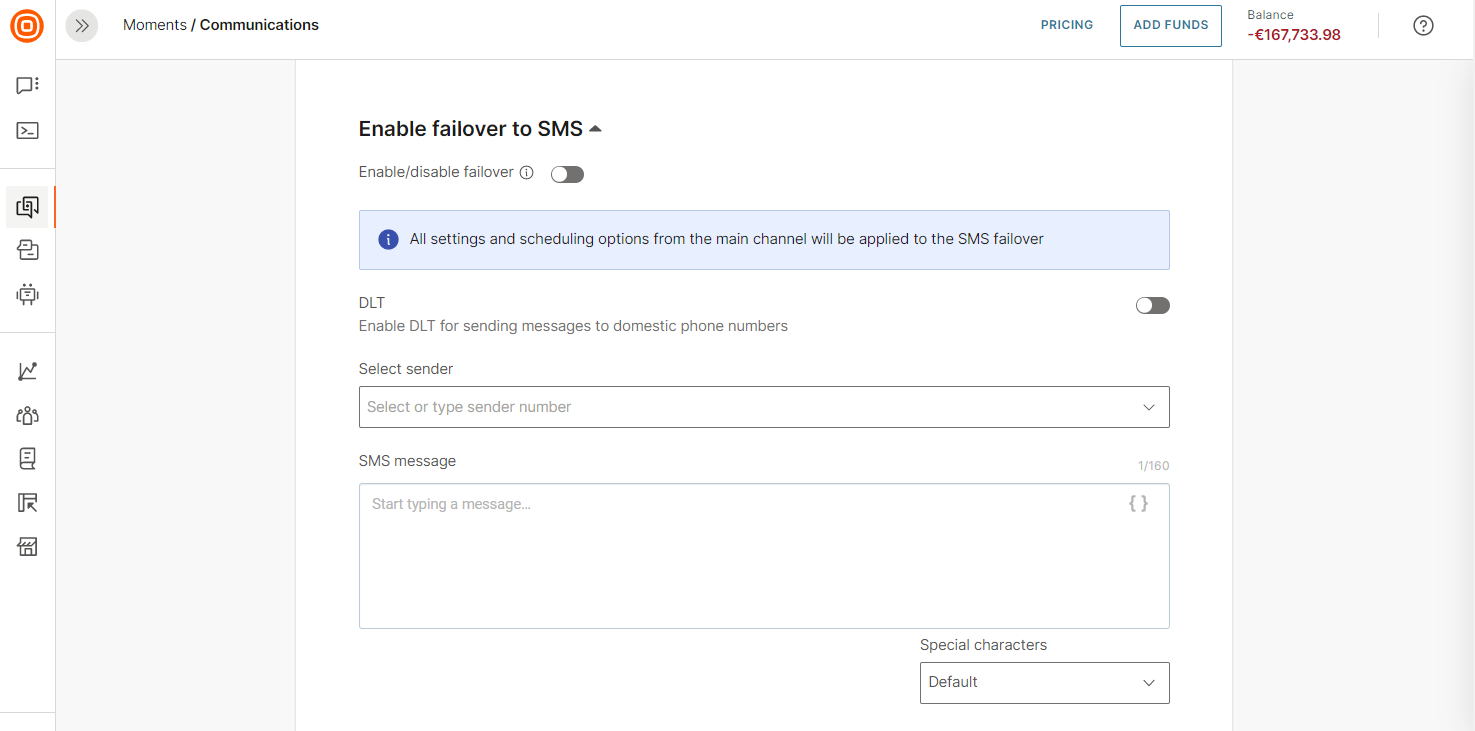The image showcases a settings interface focused on managing communication preferences. On the upper left side of the screen, there's a label that reads "Moments / Communications." Right next to this label is a vertical menu that features only symbols. At the top of this vertical menu is a distinctive logo – a series of white concentric circles within a larger red circle, giving it a resemblance to a target, with the center possibly being a square.

The main section of the interface occupies the right side of the screen, designed to display settings relevant to the selected menu item on the left. The current page is titled "Enable Failover to SMS." Beneath this title, there's an option to toggle the failover feature on or off; currently, it is toggled off. Directly below this is a bar that explains, "All settings and scheduling options from the main channel will be applied to the SMS failover," which also appears to be deactivated.